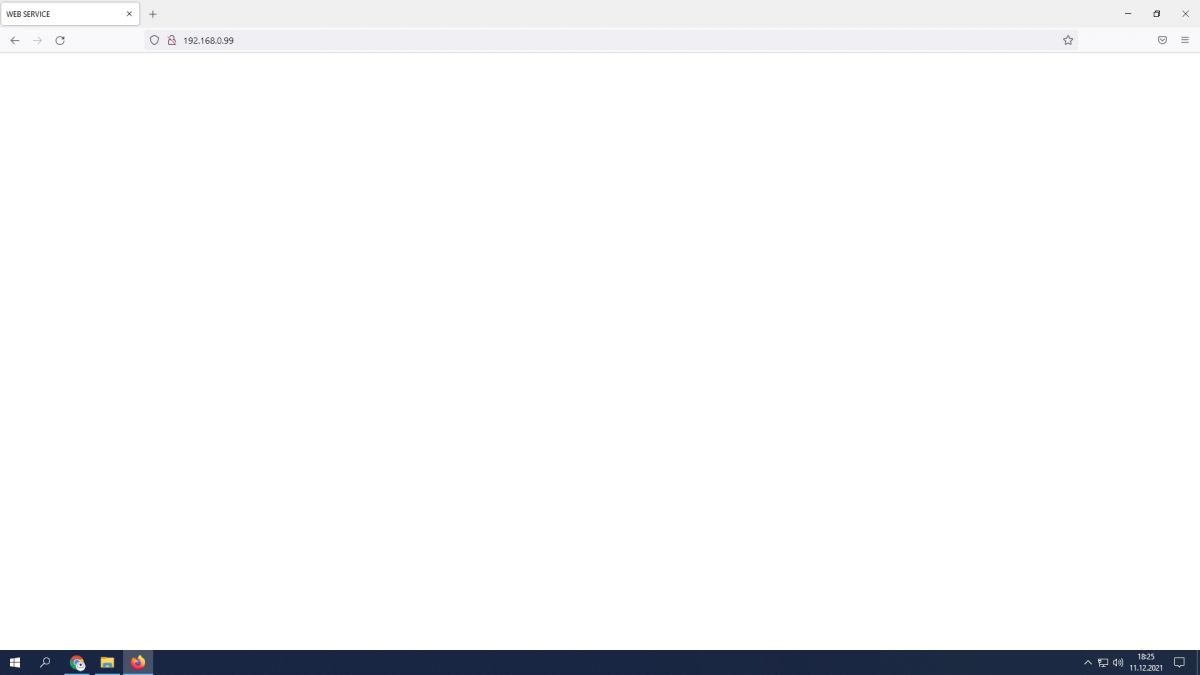This image depicts a primarily blank screen with several distinct interface elements. At the very top, there are two horizontal bars with a light gray background. The first bar contains a search box that includes a drop-down menu and options on the far right to mark it as a favorite or to exit. Below this, the second bar features left and right arrow keys, a home button, and what appears to be an IP address displayed as 192.168.399. On the far right of this bar, there are icons for exiting and returning to the home screen.

The central area of the image is predominantly blank, consisting of a white background with no additional content or elements.

At the very bottom of the screen, a black horizontal bar hosts several icons that are reminiscent of an Internet Explorer interface. On the left side of this bar, there are icons for email, search, a window, and a download or file management function. To the right, the bar displays the time, date, and settings options.